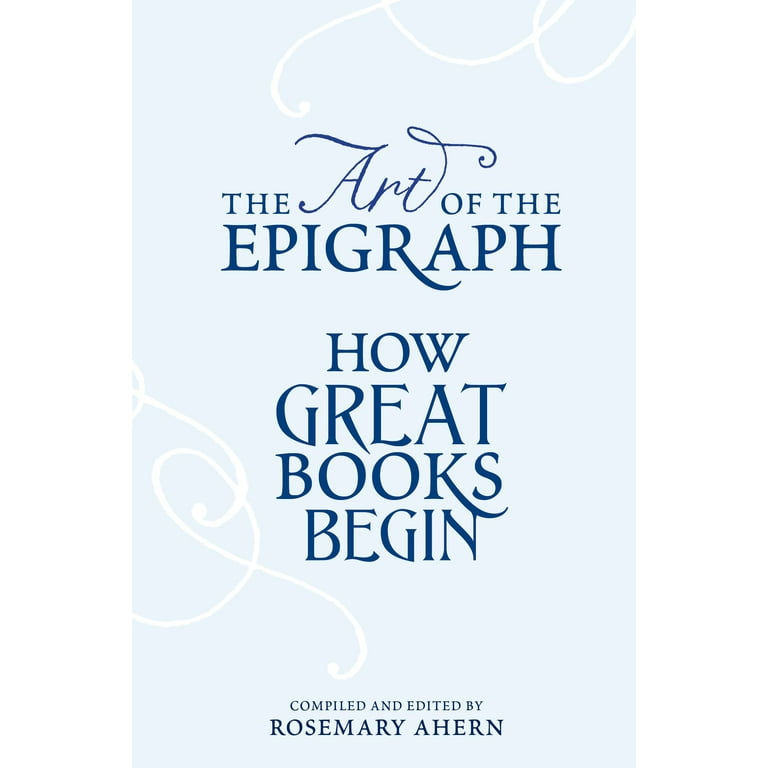This is a picture of a book cover titled "The Art of the Epigraph: How Great Books Begin," compiled and edited by Rosemary Ahern. The cover features a very light blue background adorned with elegant white, calligraphic-like squiggly patterns on the lower left and upper right corners. These decorative elements add a touch of sophistication to the design. The title "The Art of the Epigraph" is written with the word "Art" in cursive, while the rest of the words are in a standard, dark blue font. The subtitle "How Great Books Begin" is placed beneath the title, with each word on a separate line, also in dark blue. At the very bottom of the cover, the text "compiled and edited by Rosemary Ahern" is written in smaller dark blue font. The overall arrangement utilizes different font styles and sizes, lending a distinctive, eye-catching appeal to the cover.